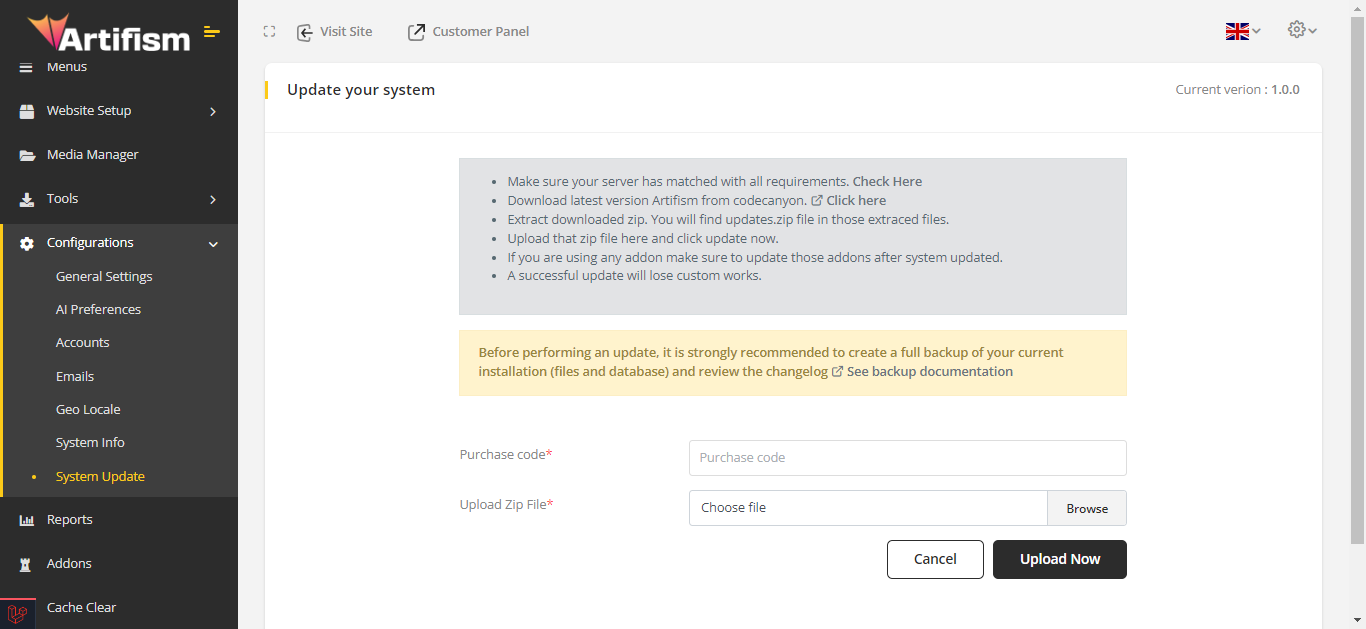The screenshot depicts a website or software interface named "Artifism," identifiable by its logo, which features a downward-facing kite adjacent to the letter "A." The image is partitioned into two distinct sections. 

On the left, occupying approximately one-fifth of the page, is a dark brown vertical background. This menu panel lists various functions including "Website Setup," "Media Manager," "Tools," "Configuration," "Reports," "Add-Ons," and a "Clear Cache" button at the bottom.

The larger, right section has a white background prominently displaying a system update notification. Central to this area is a gray rectangle with a sequence of directives, which include: "Make sure your server has met all requirements," "Click here," "Download latest version," "Extract downloaded zip," "Load that zip," and a caution that "a successful update will lose custom works."

Beneath these instructions is a conspicuous yellow rectangle advising users of the importance of creating a full backup before proceeding with the update.